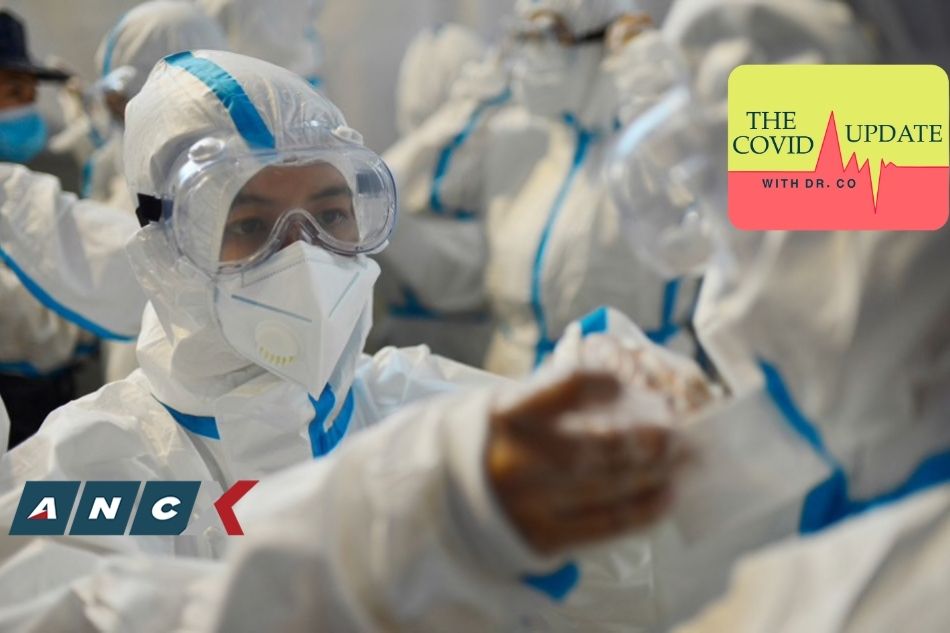This horizontally oriented photograph captures a group of healthcare or laboratory workers clad in protective gear, performing their duties amidst the COVID-19 pandemic. In the foreground, a worker is prominently featured, donning thick plastic goggles, a white face mask, and a gray plastic uniform accented with blue stripes. They wear gloves and appear to be engaged in packaging or handling materials critical to their work environment. In the background, additional workers can be seen, similarly dressed in identical protective gear, suggesting a coordinated team effort.

Distinct graphical elements frame this image: in the bottom left-hand corner, three blue rhombic icons each contain a white letter—A, N, and C—with a small triangle adjacent to the letter A. To the right of these rhombi, a red arrow points leftward. In the top right-hand corner of the image, a rounded rectangular box features a yellow top band and an orange bottom band. It displays the text "COVID Update" in black at the top, with "doctor.co" beneath it, accompanied by an image resembling a heart rate monitor line.